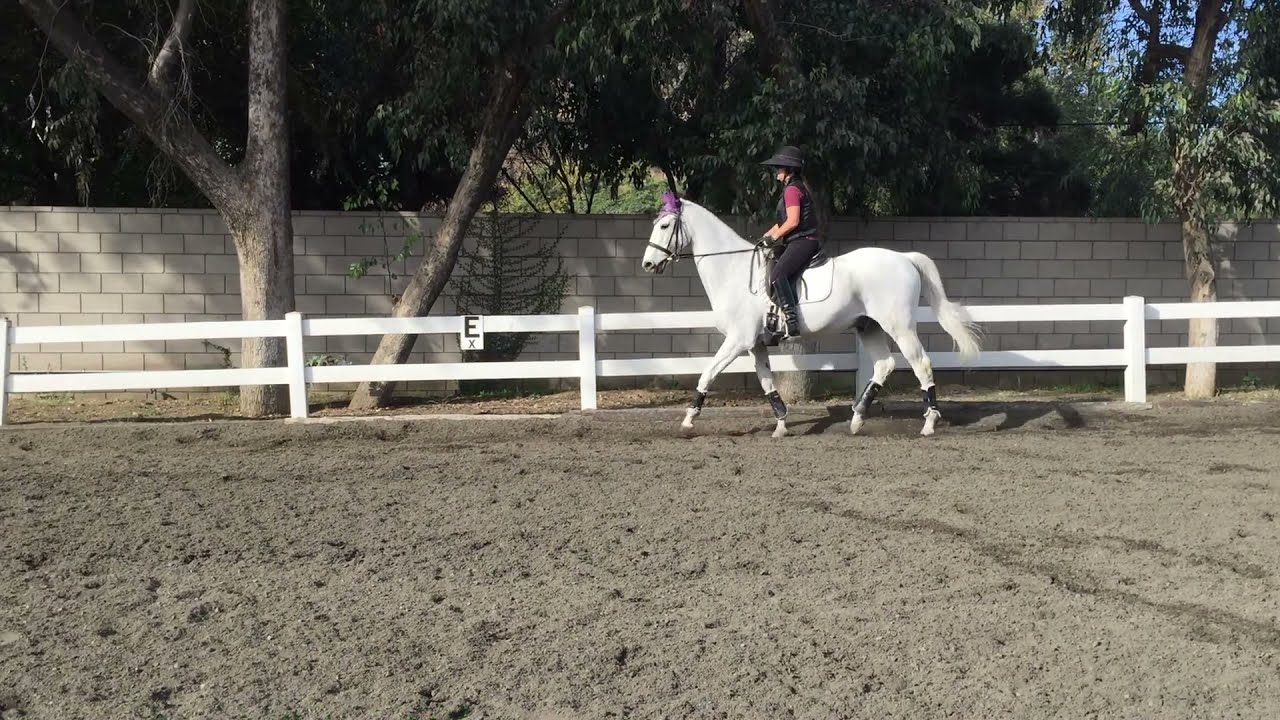This photograph captures an outdoor scene featuring a rider on a shiny white horse. The horse, oriented to the left, is adorned with a black saddle over white padding and a harness with a hint of purple near the ears. Additionally, the horse has black protective tape around its ankles. The rider is dressed in black pants and a black vest over a short-sleeved purple top, topped off with a black hat. They are situated in a dirt field, which occupies the lower portion of the image, providing a soft, grayish surface.

The backdrop includes a simple white wooden fence with vertical posts and two horizontal slats, running across the center of the photograph. An "E" and a smaller "X" can be seen on a sign affixed to one section of the fence. Beyond the fence, there is a large gray stone wall, partially obscured by lush trees that span the upper part of the image. Green foliage interspersed with patches of blue sky further enhances the natural, daytime setting.